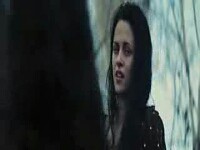In a small, cropped image that closely resembles a movie scene, a young woman appears from the shoulders up on the right side of the frame, her long, straight, dark hair either loose or obscured by a hooded jacket or sweater. Her outfit is dark, possibly black, and may feature white sequins on the left shoulder. The left side of the image is consumed by blackness, perhaps due to a nearby tree trunk or wall. The background suggests a cold, possibly snowy environment with sparse tree branches indicating a late fall or winter setting. The woman's face, turned slightly toward the camera, conveys a complex mixture of emotions—potentially confusion, sadness, or coldness—as she gazes downward, her mouth open but unsmiling. She appears to be quite young, around 20 years old, and the overall scene hints at a dramatic or melancholic narrative.